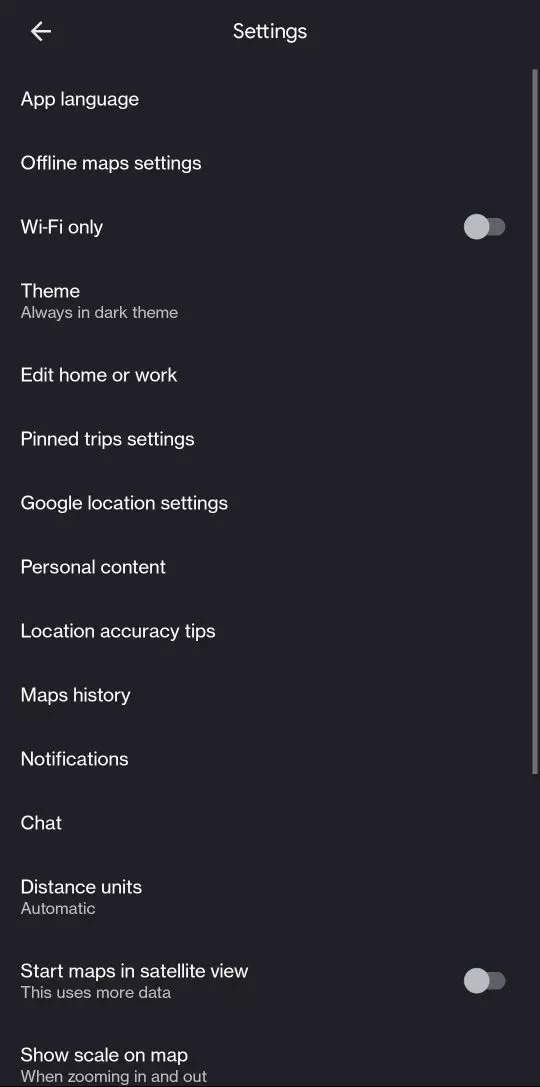The screenshot showcases a smartphone settings page with a black background. At the top of the screen, "Settings" is prominently displayed in white font, flanked by a white left-pointing arrow on the left side. Below this header, a detailed list of settings options is arranged vertically, each item also in white font.

- **App Language**
- **Offline Map Settings**
- **Wi-Fi Only**: Accompanied by a gray circle indicating that this setting is turned off.
- **Theme**: Described as "Always in dark theme".
- **Edit Home or Work**
- **Pinned Trip Settings**
- **Google Location Settings**
- **Personal Content**
- **Location Accuracy Tips**
- **Maps History**
- **Notifications**
- **Chat**
- **Distance Units**: Displayed with a subtext "Automatic".
- **Start Maps in Satellite View**: This setting is turned off, denoted by the gray circle, with an additional note mentioning "This uses more data."
- **Show Scale on Map**: With a subtext "When zooming in and out."

This descriptive outline details each specific setting visible in the screenshot, capturing the visual and functional elements of the smartphone's settings page.